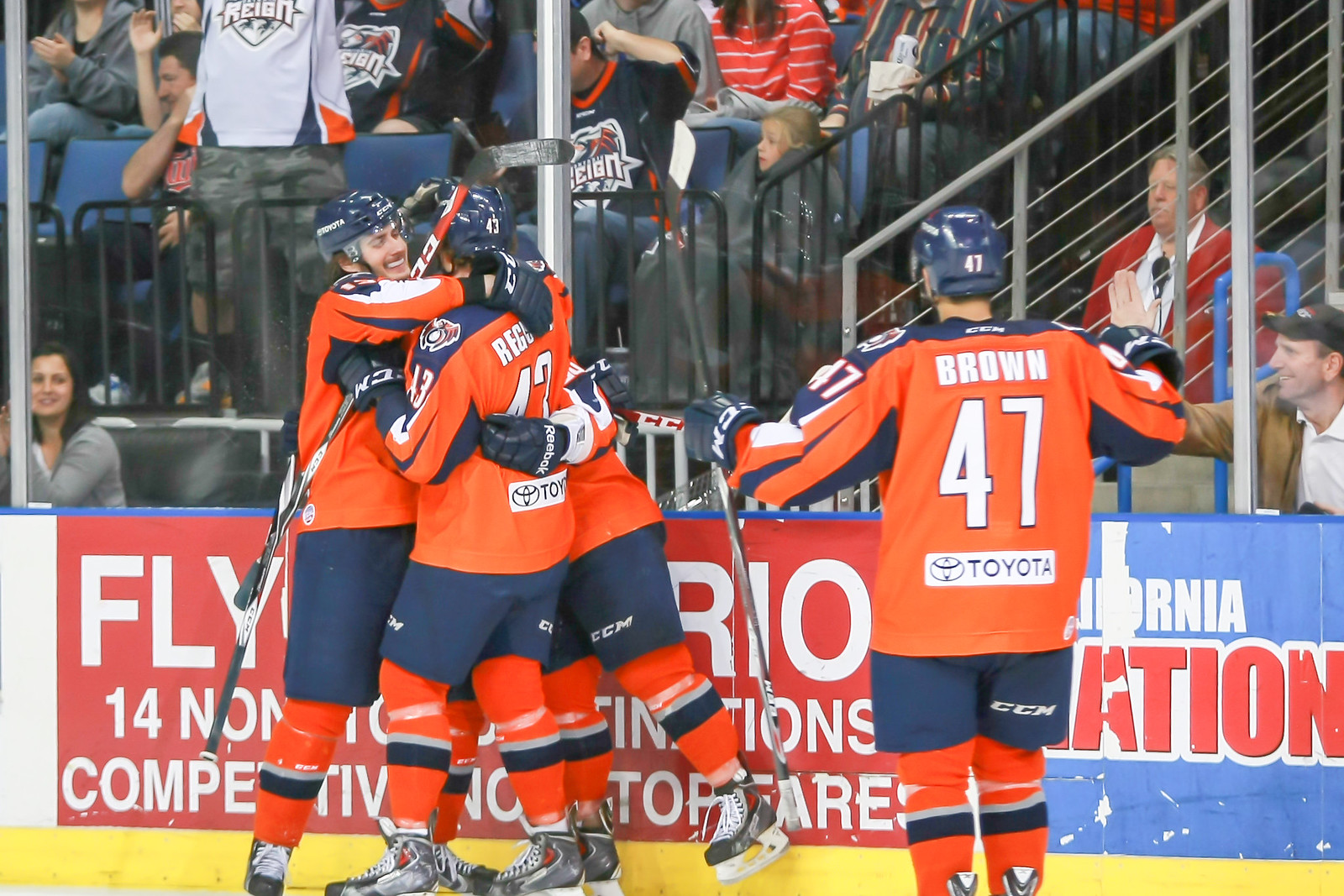In the image, a lively ice hockey scene unfolds within an indoor stadium. At the heart of the photo, three ice hockey players are enthusiastically celebrating near the boundary of the rink, warmly embracing each other. They are donned in striking orange jerseys with blue shoulders, white numbers, and a Toyota logo at the back, complemented by blue half-pants, orange socks, and gray skates. A fourth player, with "Brown 47 Toyota" inscribed on his back, is skating towards them, holding a hockey stick.

Surrounding the rink, a solid pane of glass separates the players from the audience. Beyond this barrier, spectators are seated, attentively watching the celebration through the transparent shield. The setting is adorned with various sponsor banners, including a prominent red banner on the left and a blue one on the right, mounted against a white wall. Below the banners, behind black barricades and alongside stairs leading to an upper level, the fans contribute to the vibrant atmosphere of this moment captured during the game. The indoor arena is filled with colors that highlight the dynamic nature of the scene, featuring hues of white, red, yellow, blue, orange, black, and gray.